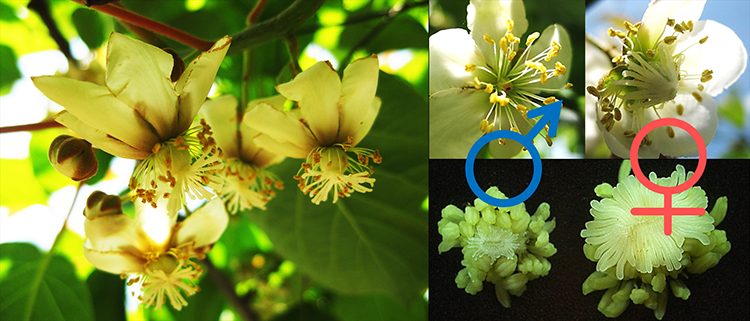The photograph is a detailed botanical collage featuring images of flowers in various stages and close-ups. The left side of the collage showcases a larger photograph of a tree branch adorned with clusters of white flowers, each consisting of about four individual flowers and two buds. The flowers are characterized by white petals with brown centers and brown parts. Yellowish leaves serve as the backdrop, indicating the picture was taken outside in sunlight.

On the right side, the collage is divided into four evenly spaced rectangular photographs. The top sections feature close-up images of white flowers with cream-colored petals and long stamens tipped with yellow points. The petals point upward, and the stamens extend outward. The close-up images distinguish between male and female flowers using blue and red symbols respectively, indicating gender differences.

The bottom left corner features a detailed close-up of the flower’s reproductive system on a black background, emphasizing the distinctive parts of the flowers. The collage provides an educational insight into the flowers, with a clear botanical theme illustrating different parts and stages of the flowers, as well as their gender differentiation.